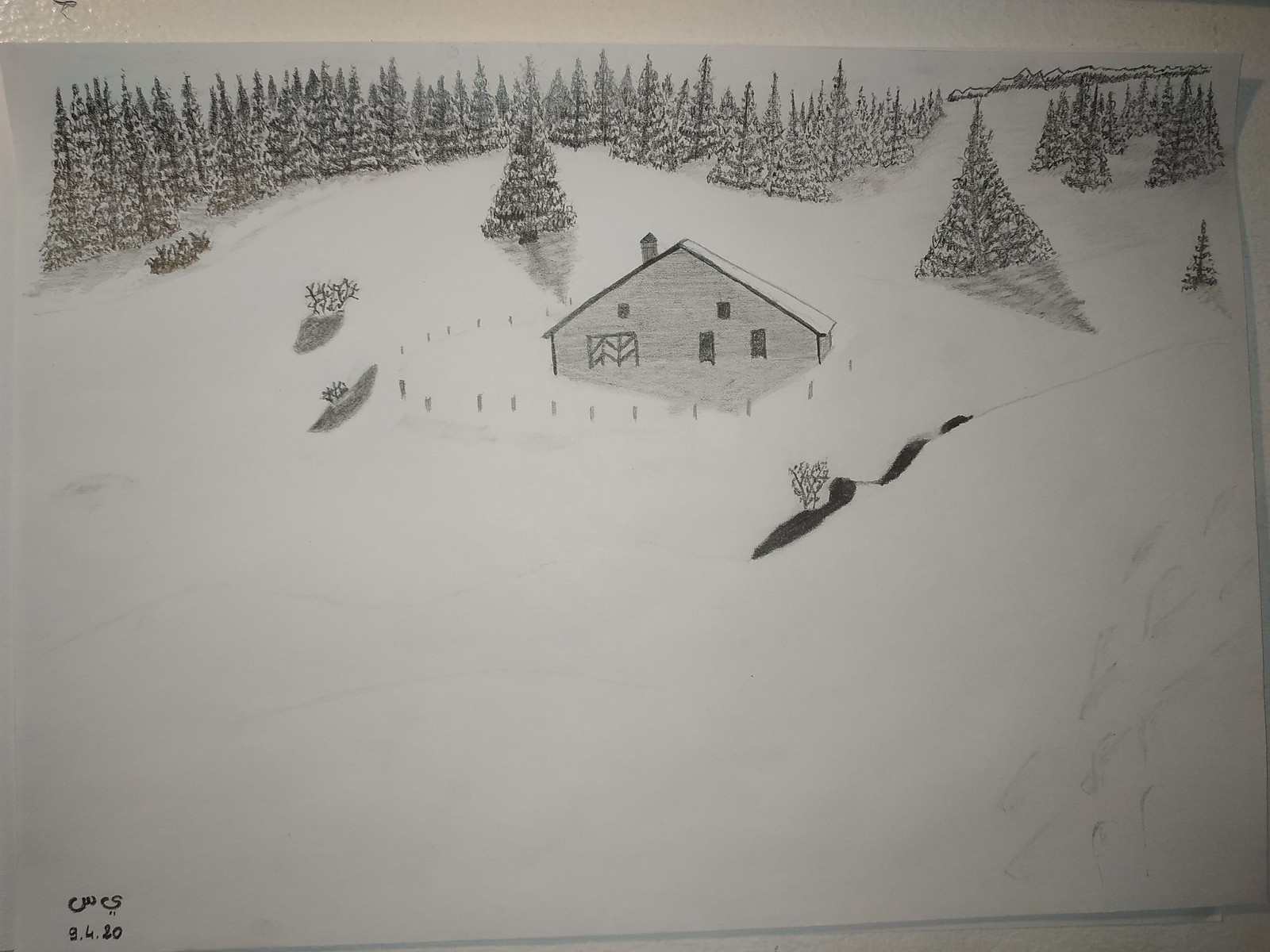A detailed pencil or charcoal illustration depicts a serene winter landscape. The background features a dense forest of Christmas tree-like evergreens scattered predominantly across the right side of the composition. The foreground, dominated by a pristine expanse of snow, suggests a tranquil, untouched terrain. 

Centrally positioned is a modest gray house with black windows and a small chimney, surrounded by sparse, stick-like structures protruding from the ground. Flanking the house on both the left and right sides are small, grayish-black mounds adorned with dead, barren plants, adding a somber touch to the scene.

In the bottom left corner, partially legible black writing is accompanied by a date that appears to read "9/4/80." The illustration is framed against a white surface, potentially a wall or counter, setting off the quiet, monochromatic beauty of the winter scene.